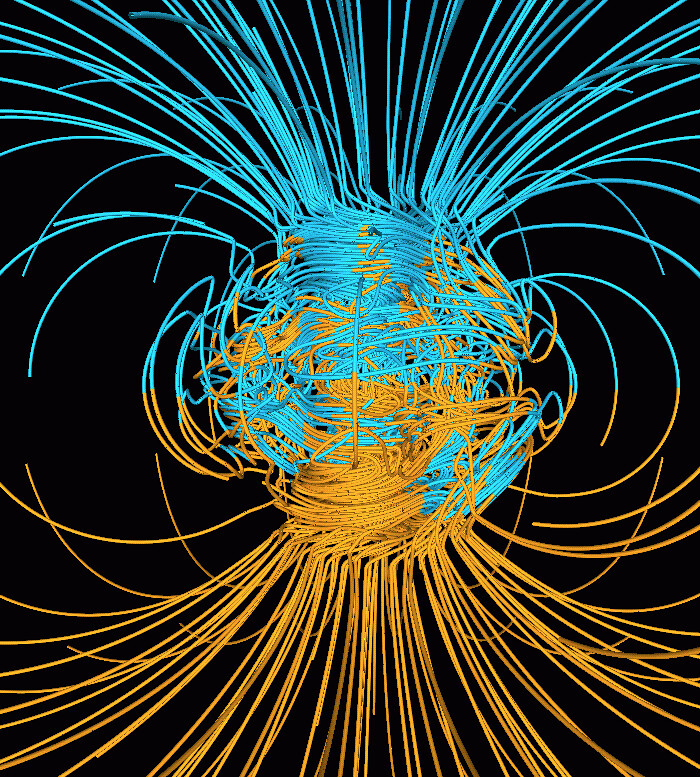The image displays a computer-generated piece of digital art against a solid black background. The focal point is a complex, large, rectangular shape dominated by intertwined strings or lines in two distinct colors: blue and yellow. At the top of the image, blue strings are more prevalent, while at the bottom, yellow strings take prominence. These strings seem to go in various directions—some straight, others slightly bent.

In the central area of the image, these blue and yellow lines intricately mix and twist together, forming a dense and tangled core. This section appears almost like a chaotic puzzle or a ball of spaghetti in a circular shape, with intertwining colors creating a striking visual contrast. The core seems to be the focal point where the lines are most densely packed.

From this tangled center, the lines extend outward. At the top, blue lines dominate, projecting both vertically and diagonally towards the upper corners. Similarly, from the bottom, yellow lines spread out, following similar projection patterns. Some lines switch their color midway, adding to the complexity, and suggesting a continuous interaction between the colors. The bottom portion of the circular tangle has a concentration of yellow, while the upper part leans towards blue, with some streaks of yellow mingling in.

Overall, the image evokes an abstract and dynamic feel, emphasizing the central mass of intertwined lines as the strongest point, with the strings extending outward in a balanced but intricate fashion, likely created through sophisticated digital art software.